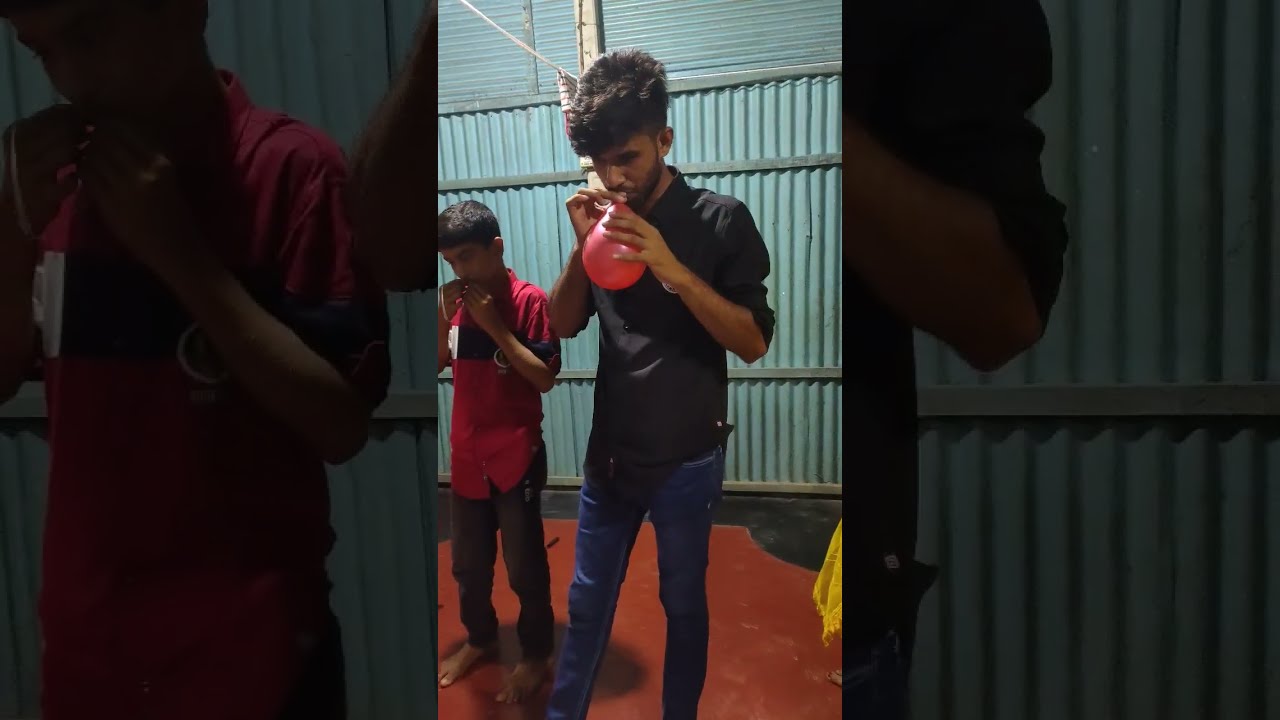The image is a vertically-oriented cellphone photo depicting two individuals of likely Indian descent, standing outdoors on a red-and-black painted cement surface. The man on the right, slightly taller with thick brown hair, is wearing a black shirt with its sleeves scrunched up and blue jeans. He is in the process of blowing up a red balloon. Next to him, on the left, is a barefoot younger boy with short dark hair, clad in a red polo shirt featuring a blue stripe and black pants, with his hands near his mouth, possibly blowing a balloon as well. Behind the pair stands a light blue, corrugated metal wall, extending up to a sloping roof of the same color. Situated in front of the wall, an electrical pole with a low-hanging wire is visible. Additionally, the bottom right corner of the image reveals part of a yellow "wet floor" sign, despite no corresponding wet floor. The photo itself is framed by a faded, zoomed-in version of the same image on either side.